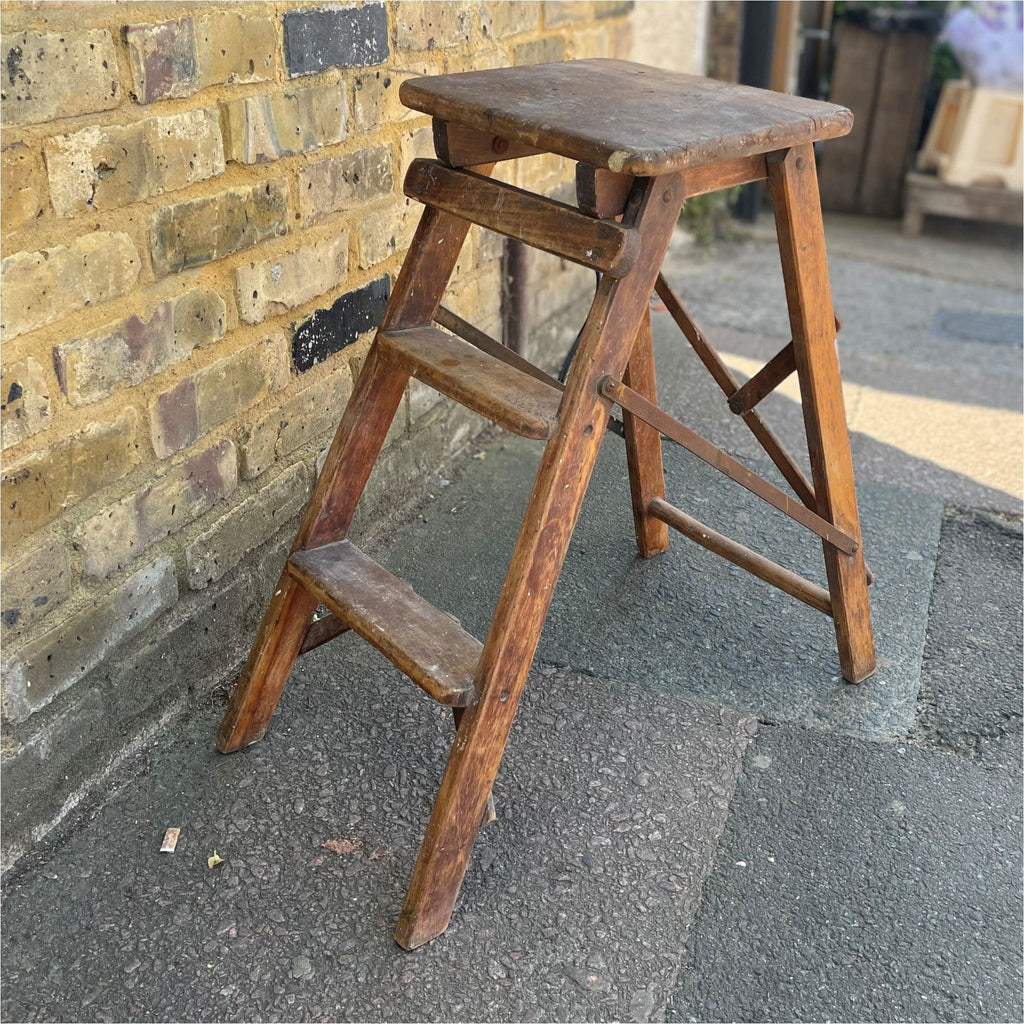This is an image of an old, wooden step stool that appears well-worn and weathered from years of use. The step stool, which seems to be a walnut-stained wood, features two main steps in the front and a flat top surface for stepping. There's notable dust, chips, and remnants of paint indicating it's an earlier model, with stained hardware connecting the folding front to the back legs. The stool appears somewhat rickety and not sturdily built, suggesting limited support capacity.

The step stool is positioned outside on a gray stone pavement consisting of large squares of cement. It is set against a distinctive brick wall composed of light beige and red bricks, accented with occasional black bricks. The wall's bricks also display varying shades of purple, gray, and tan. In the background, a wooden door or fence and a pile of assorted objects can be seen.